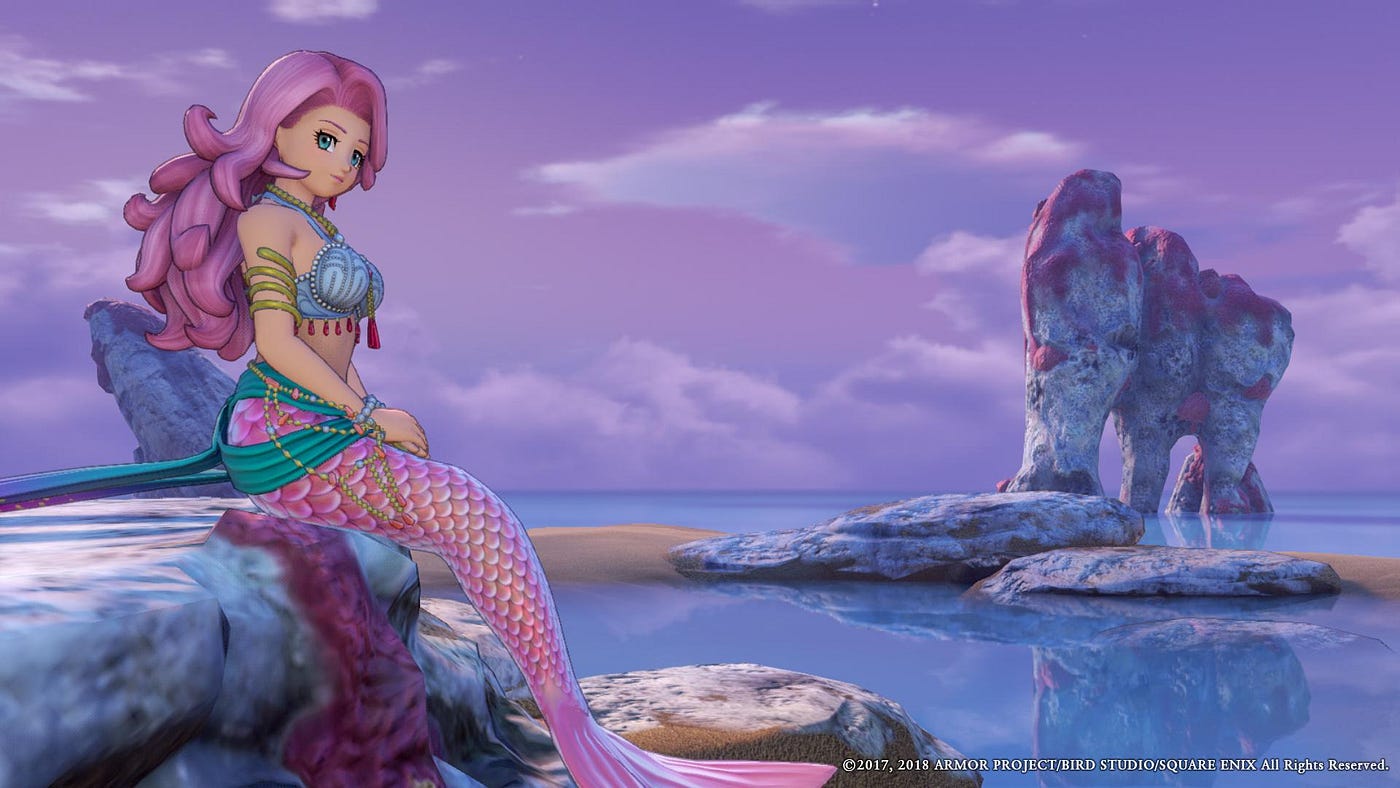In this vibrant screenshot from a video game, the scene bursts with bright and vivid colors dominated by blues, pinks, and purples. The background features a fantastical, cloudy sky drenched in purple hues, adding to the dreamy atmosphere. On the left-hand side, a captivating mermaid character is seated gracefully on a rock. She has long, fluffy pink hair cascading down her back, adorned with a golden armband. Her attire includes a turquoise shawl wrapped around her waist, a light blue or gray top with red tassels, and, of course, her striking pink-scaled tail. The surrounding water is speckled with stones, and a rocky, three-pronged mountain rises majestically from it, detailed with white, gray, and hints of purple moss. The image, rich with digital artistry and 3D graphics, bears the text "Copyright 2017-2018 Armor Project/Bird Studio/Square Enix. All rights reserved" in the bottom right corner, affirming its creative origins.